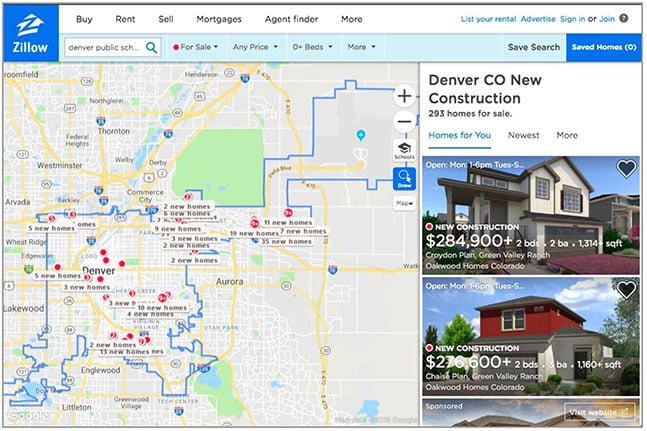This screenshot captures the user interface of Zillow, specifically focusing on the search results for homes in the Denver Public Schools area. A black and light gray border frames the entire screenshot for emphasis. In the upper left-hand corner, the prominently displayed Zillow logo is accompanied by several navigation tabs: Buy, Rent, Sell, Mortgages, Agent Finder, and More. The upper right-hand corner features actionable blue links: List Your Rental, Advertise, Sign In, or Join. 

Directly below these links, a light blue background houses a search bar where the user has entered "Denver Public Schools" along with the condition set to "For Sale." The search filter settings include "Any Price" and "0+ Beds," with additional options available under "More." There is also a button to save the search criteria for future reference.

On the right-hand column of the interface, the results are shown, starting with a header that reads "Denver, Colorado, New Construction, 293 homes for sale." Below this, individual listings begin with an entry for a home priced at $284,900 featuring 2 beds and 2 baths in the Croydon Plan, followed by another new construction listing priced at $276,600. 

At the bottom right corner, a partially visible sponsor label indicates that the image has been cut off, suggesting that the user was scrolling through the search results when the screenshot was taken. On the left side, a large map illustrates the Denver Public Schools area, with red dots marking the locations of homes for sale.